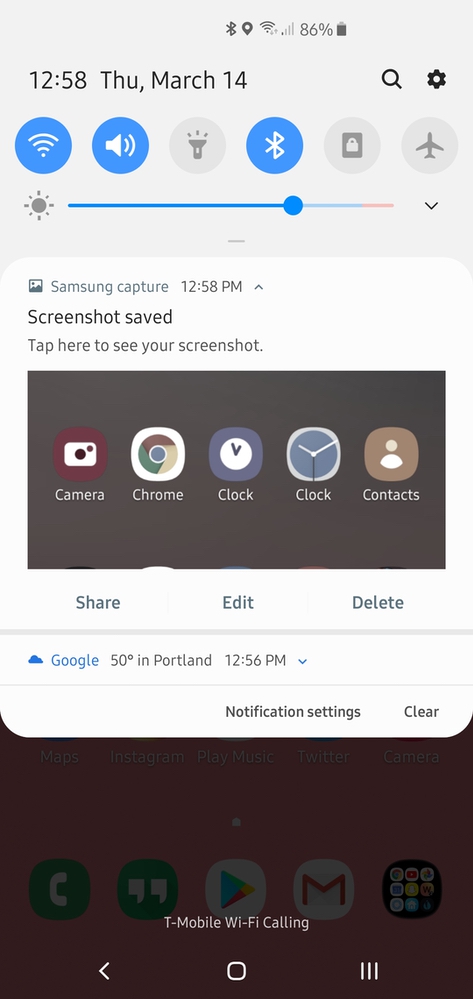A screenshot of a smartphone's home screen reveals various interface details. At the top of the screen, there's a white status bar displaying the Bluetooth icon, location services, Wi-Fi signal strength, cellular signal (with only one bar lit), and an 86% battery level. Just below this, in a larger font, it indicates the time as 12:58 PM and the date as Thursday, March 14th. On the right side, there are icons for search (a magnifying glass) and settings (a gear).

Directly beneath the date and time is a row of six circular icons: Wi-Fi, sound, flashlight, Bluetooth, screen lock, and airplane mode. Among these, the Wi-Fi, sound, and Bluetooth icons are illuminated in blue, indicating they are active. Adjacent to these circles is a brightness slider, which is mostly filled, suggesting high screen brightness.

Further down, a notification from "Samsung Capture" states a screenshot was saved at 12:58 PM, with options to tap and view. Below this notification is a black box featuring icons for Camera, Chrome, Clock, and Contacts, with an additional row below that providing options to share, edit, or delete the screenshot.

Continuing lower, a Google weather update states it's 50 degrees in Portland at 12:56 PM, with a downward arrow for additional options. The notification bar offers choices for notification settings and clearing all notifications.

The lower segment of the screen, showing a darkened or grayed-out home screen, includes app shortcuts at the very bottom for Phone, Chrome, Gmail, and a general Apps button. The text "T-Mobile Wi-Fi calling" appears near the bottom, alongside the navigation bar with a back button.